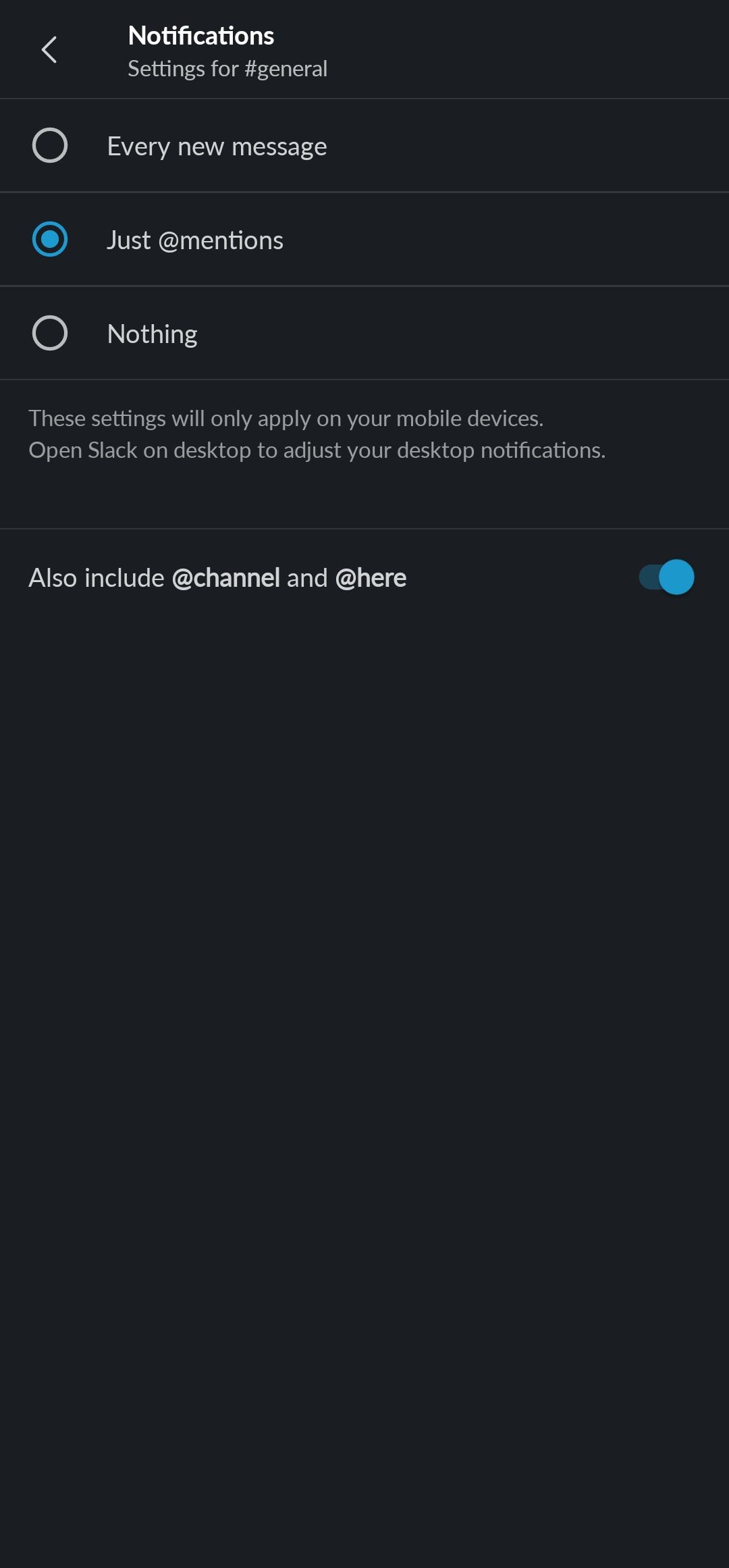This is a screen capture of a notification settings window on a black cell phone screen within the Slack application. 

- At the top-left corner, there is a left-facing triangle icon representing a back arrow.
- Next to the icon, in bold white text, it says "Notifications". 
- Underneath "Notifications", in a lighter white font, it reads “Settings for Pound General”.

Following this header, there is a light-colored horizontal gray line.

Underneath the gray line:
- It says "Every New Message" in white lettering.
- To the left of this text, there is an unchecked white radio button.

Below another horizontal gray line:
- It reads "Just Add Mentions" in bold white letters.
- To the left of this option, there is a turquoise blue radio button, indicating it is selected.

Further down, below an additional gray line:
- The word "Nothing" appears in white text.
- To the left of this, there is another white radio button that remains unchecked.

Below another gray line:
- Light white text indicates: "These settings will only apply on your mobile devices. Open Slack on desktop to adjust your desktop notifications."

At the bottom line, in dark, bold white text, it states:
- "Also include @channel and @here".
- To the right of this text, an oval slide button is shown in which a turquoise-colored blue circle is slid to the right-hand side, signifying that the option is turned on.